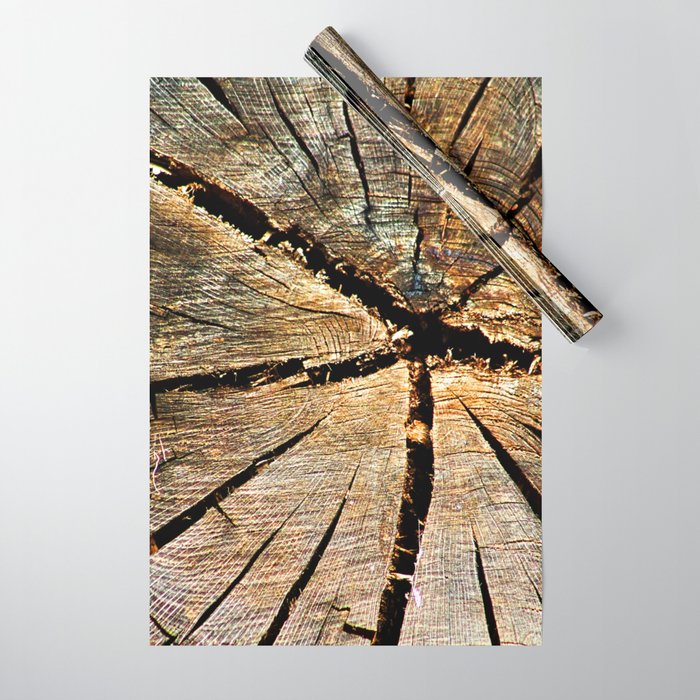The image displays a detailed, close-up view of a tree trunk, captured from above, showcasing its natural aging process and intricate splits radiating from the center. The tree trunk dominates the rectangular frame, with its dark orange core gradually fading to lighter brown shades at the top and bottom. The surface features natural wood tones and darker shading in the eroded and cracked areas. The background surrounding the tree trunk is a light gray color, which contrasts with the wooden textures. Lying across the upper right corner of the trunk is a cylindrical object, resembling a scroll, that shares the same textured wood appearance and color palette, as if it were another piece of the tree trunk itself. This detailed composition emphasizes the organic beauty and complexity of the tree’s surface.